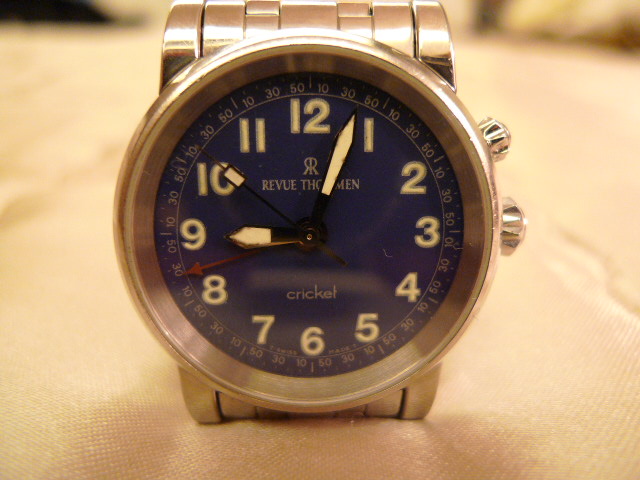The image showcases a shiny, stainless steel analog wristwatch positioned centrally on a soft yellow fabric. The watch features a sleek, gold-colored chain wristband and a circular gold case. On the right side of the watch, there are two rotary dials, also gold in color, used for adjusting the time. The face of the watch, under the glass, is a dark blue with white text. 

The dial displays the numbers 1 to 12 in white, with the 12, 3, 6, and 9 prominently marked. Surrounding these numbers is an outer ring with seconds demarcated in intervals of 10, 30, and 50. The inner dial also contains words such as "Review," "Dorman," and "Cricket." 

The watch has four hands: the hour hand, which is black and white and currently pointing at 9; the minute hand, also black and white, positioned between 12 and 1; the red hand, which appears to be a chronograph hand, pointing between 8 and 9; and a skinny black second hand with a white tip, positioned at 10. The overall appearance of the watch is highly polished and metallic, with its design emphasizing both functionality and elegance.